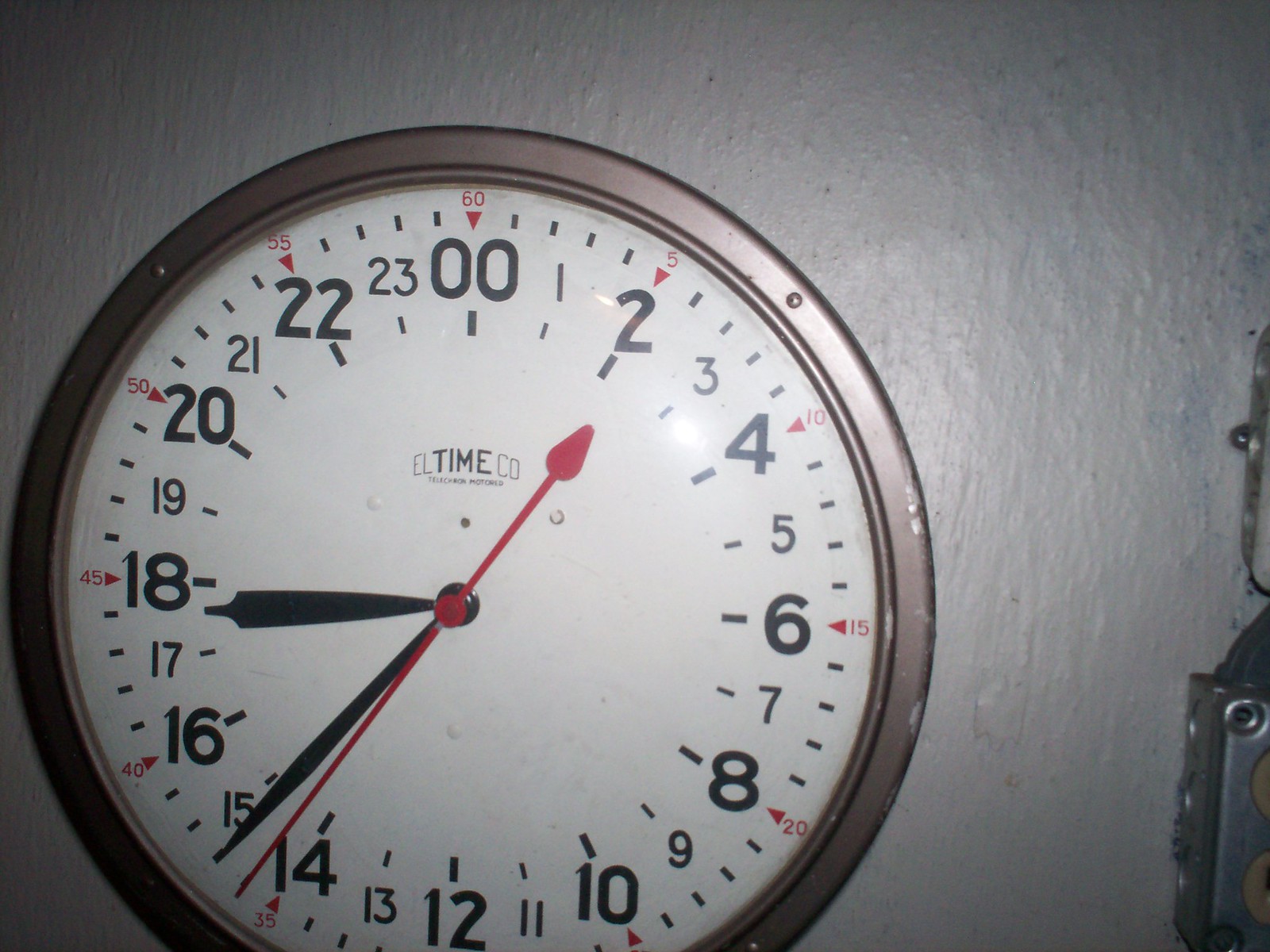In the image, there is a textured gray wall reflecting light. Mounted on the wall is a round military clock, displaying time in a 24-hour format. The clock, which reads approximately 08:35, features black numerals ranging from 00 to 23 with small red triangles at the positions of 00 and 02. The clock face is white and prominently displays the logo "Time Co" in the center. The clock is encased in a wooden-rimmed border, adding a warm contrast to the gray wall and white dial.